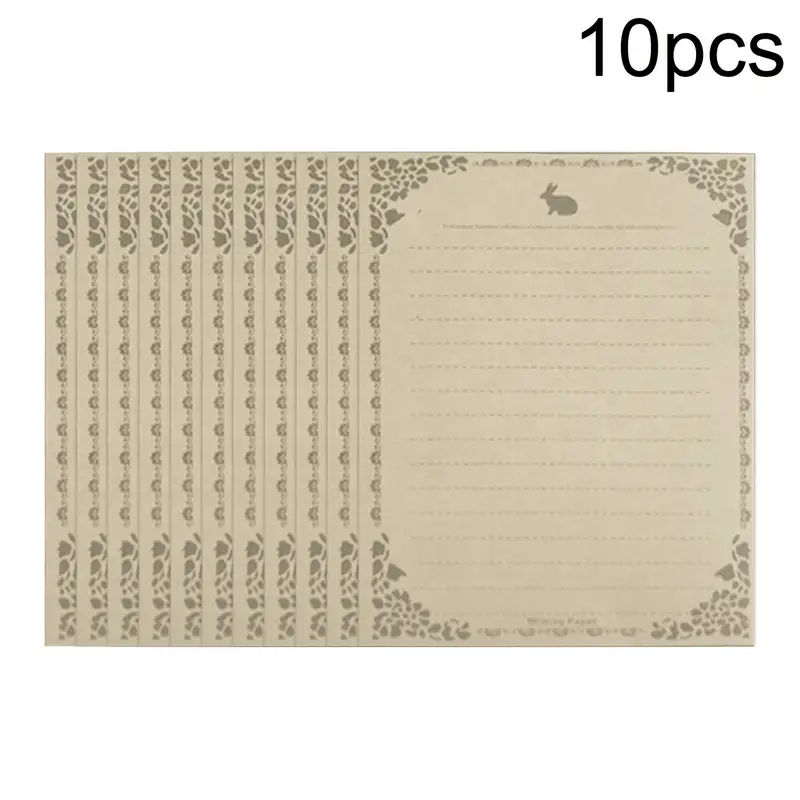The image features a horizontally aligned rectangular photograph showcasing a set of 10 pieces of blank stationery against a white background. Each sheet is a vertical rectangle, predominated by a light taupe color. The top center of each sheet is adorned with a shaded gray silhouette of a bunny facing left, positioned prominently where the letterhead would be. Beneath the bunny image, dashed lines run vertically down the page, intended for writing. The sheets are fanned out slightly to the left, revealing just the left edge of each overlapping sheet, creating a layered effect. The edges of the paper are framed with a border of irregularly shaped, gray-shaded designs reminiscent of leaves or flowers, thickening at the corners. At the upper right corner of the image, "10 PCS" is prominently displayed in large black text, indicating the quantity of the stationery set.